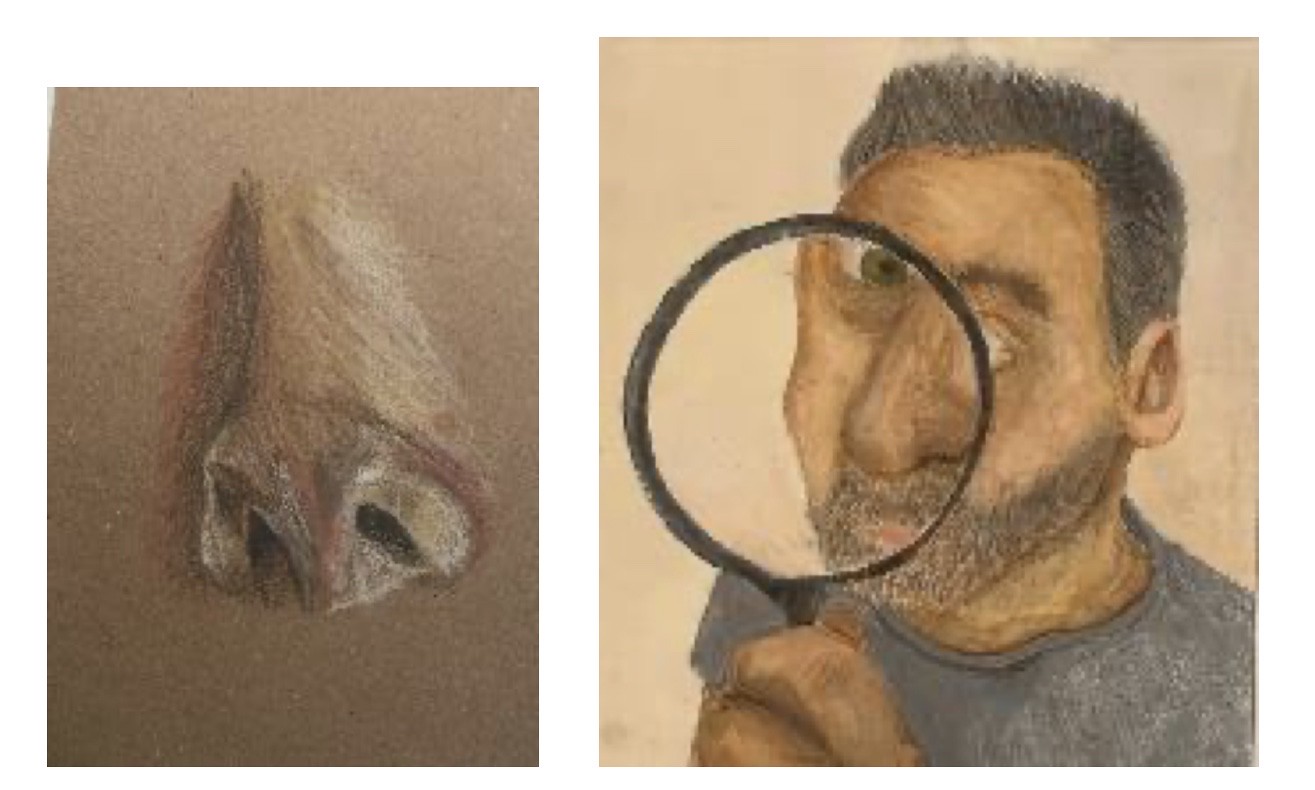A very poorly executed chalk sketch depicts a man examining himself through a magnifying glass. The figure appears skewed and distorted, particularly the details seen through the magnifying glass. The man, who has short, somewhat spiky hair with a receding hairline and a dark complexion, looks unkempt with a few days' worth of stubble. He's holding the magnifying glass in his left hand, which expands his eye, nose, part of his lips, and cheek to exaggerated proportions, albeit inaccurately placed. He is dressed in a gray shirt. To the left of the main figure, there is an additional image of a nose that seems deformed—resembling either a non-human nose or the result of botched plastic surgery, with misshapen, bruised nostrils. The purpose of the drawing is unclear, and overall, the execution is subpar.